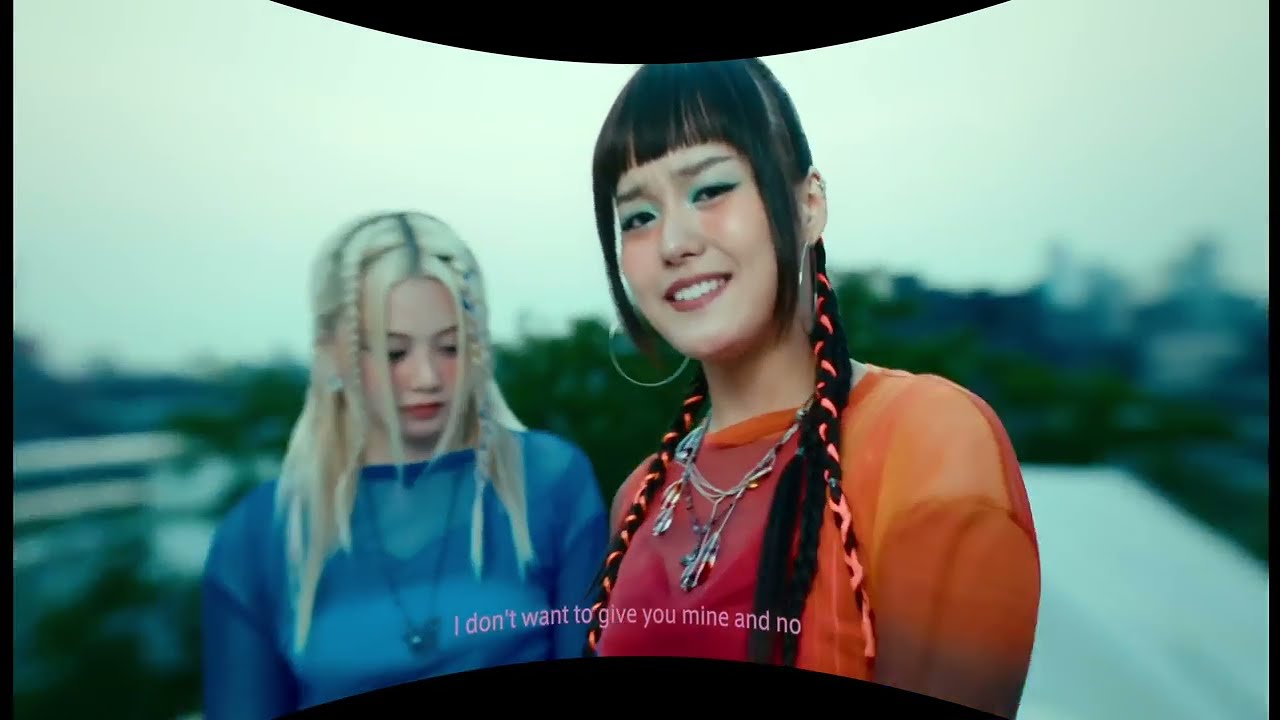In this image, we see two young women, both of whom appear to be of Asian descent, standing together in an outdoor setting with a blurry background consisting of a white sky and green trees. The photograph has a fisheye or VR effect, making the edges bow inward at the top and bottom.

The woman in the center is wearing an orange long-sleeve top with a red lacy front. She has long black hair styled with braids, decorated with colored rubber bands or threads braided through. Notably, she is adorned with multiple silver chains around her neck, large hoop earrings, and blue eyeshadow. Her vibrant, red lipstick adds to her striking appearance, along with her smiling expression.

To her left stands another woman with long blonde hair, also featuring a few braids. Her hair is parted down the middle. She is dressed in a long-sleeve, lacy light blue shirt, and wears a pendant necklace. She looks slightly downward and has noticeable pink lips.

Overlaying the bottom of the image, there are subtitles that read, "I don't want to give you mine and no," suggesting that this might be a screenshot from a video featuring music lyrics.